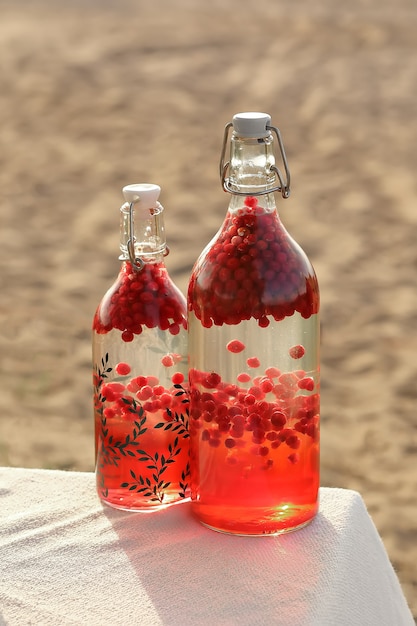This photograph, set against a blurred, sandy desert backdrop, captures two clear glass bottles positioned side by side on a white terry cloth. Both bottles are capped with white lids secured by metal fasteners and contain layered liquids. The larger bottle on the right is filled with clear liquid, in which clusters of small, round, red berries float at the top, with some gradually sinking into the liquid. These berries create a transition from clear liquid at the top to a pinkish-red, opaque liquid at the bottom. The smaller bottle on the left, featuring an etched green vine design, mirrors the same intriguing arrangement of clear liquid and descending red berries, culminating in a similar red liquid at the bottom. The overall scene evokes a stark contrast between the vibrant contents of the bottles and the muted desert environment.